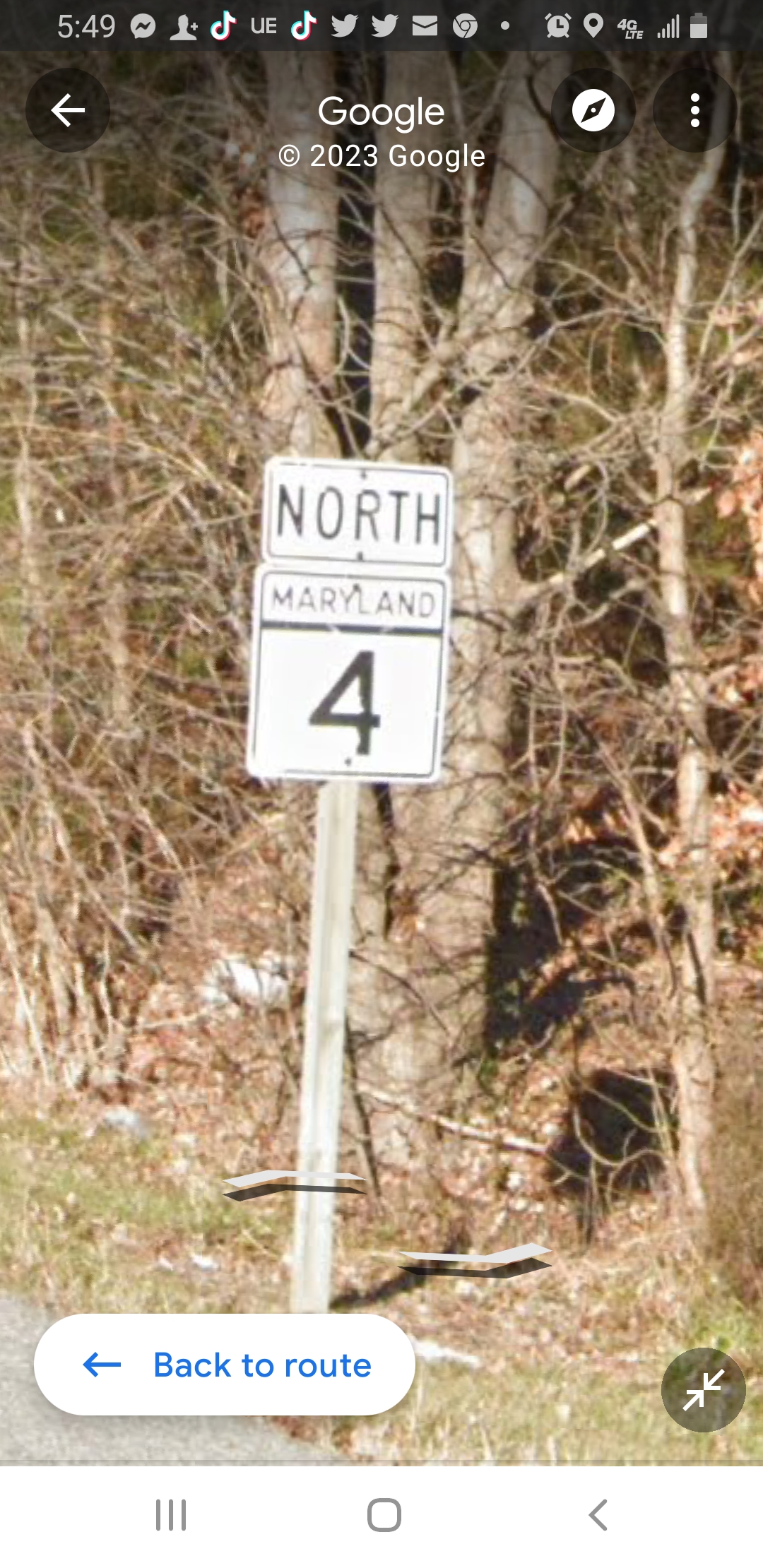This detailed caption aims to synthesize all the provided voice captions into a cohesive and comprehensive description:

---

The image is a color screenshot taken on a mobile phone, identifiable by the time "5:49" and various social media and utility icons such as Twitter and 4G LTE displayed at the top. It features a vertical, rectangular road sign situated along a tree-lined street, washed in muted brown tones with patches of grass visible at the bottom. The upper part of the road sign, mounted on a gray pole, reads "North" and directly below it is another sign stating "Maryland" with the route number "4," all framed within black square borders. At the top of the image, "Google" along with the copyright notice "© 2023 Google" is visible, indicating it likely originates from Google Maps or Google Images. Additionally, the bottom section of the screen includes interface elements: a white text box with the blue text "Back to Route" accompanied by a left-pointing blue arrow on the lower left, and a circular icon displaying two white arrows pointing toward each other on the lower right. The background is populated with trees, providing a subdued natural setting behind the road sign.